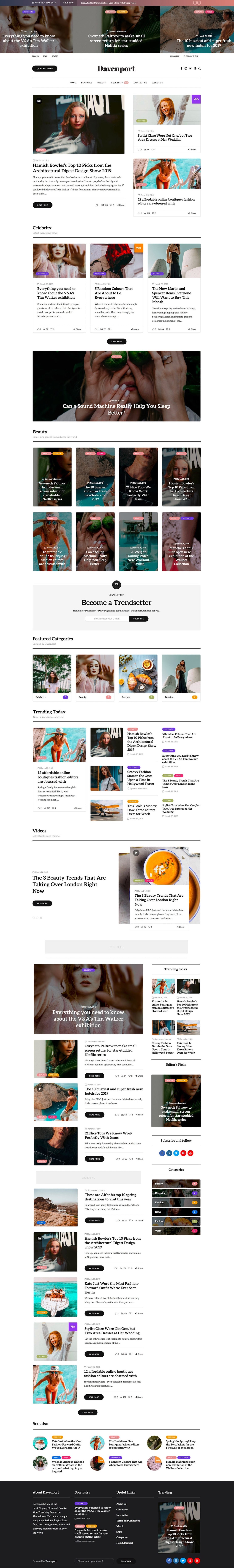This is a very blurry screenshot capturing the homepage of a website, condensed into one image. The screenshot was taken on Monday, May 8th, 2019, as noted in the top left corner. To the right, there's a section labeled "Trending," followed by a featured article titled "Groovy Fashion Stars in the 'Once Upon a Time in Hollywood' Teaser." 

At the top right of the page, two navigation buttons allow users to scroll left and right through the featured content.

The top of the homepage showcases three main articles:

1. **Left Article:**
   - **Title:** "Everything You Need to Know About the V&A's Tim Walker Exhibition"
   - **Date:** March 28th, 2019
   - **Category:** Celebrity (indicated by a filter or banner)

2. **Middle Article:**
   - **Title:** "Gwyneth Paltrow to Make Small Screen Return for Star-Studded Netflix Series"
   - **Content Type:** Sponsored Content
   - **Tags:** Beauty, Fashion

3. **Right Article:**
   - **Title:** "The 10 Buzziest and Superfresh New Hotels in 2019"
   - **Date:** March 25th, 2019
   - **Tags:** Beauty, Video

Despite the low resolution, the content and structure of the homepage are discernible, providing a glimpse into the trending topics and featured articles of that particular day.